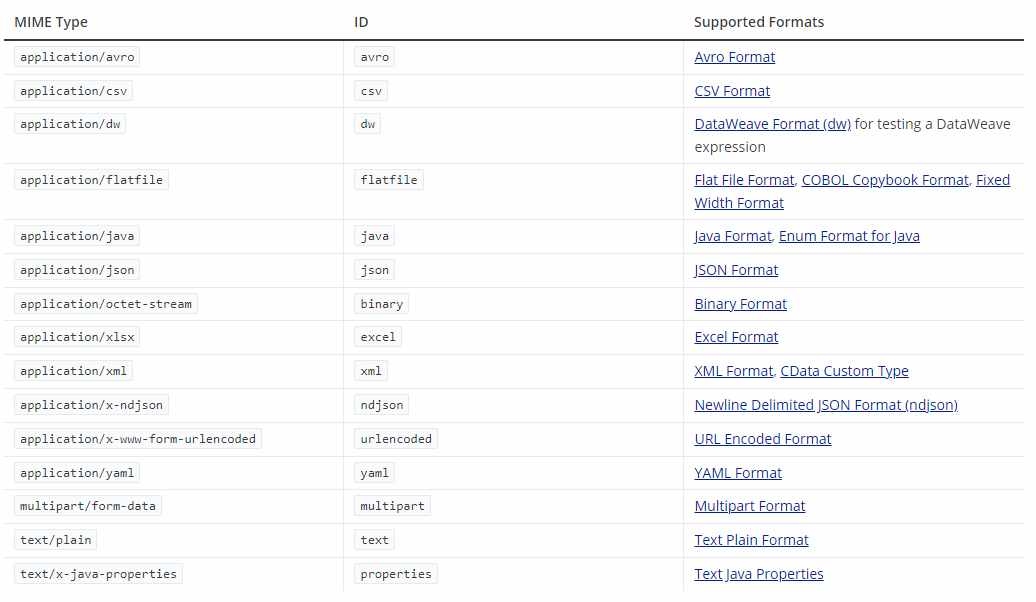Screenshot of a table with three columns: "MIME Type," "ID," and "Supported Formats." The table is organized by horizontal lines dividing each entry, with clickable links located in the "Supported Formats" column. The first row of the table features the MIME Type as "application/avro," with its corresponding ID listed as "Avro," and the Supported Formats column indicating "Avro format." The columns are clearly labeled at the top, with "MIME Type" on the left, "ID" in the middle, and "Supported Formats" on the right.